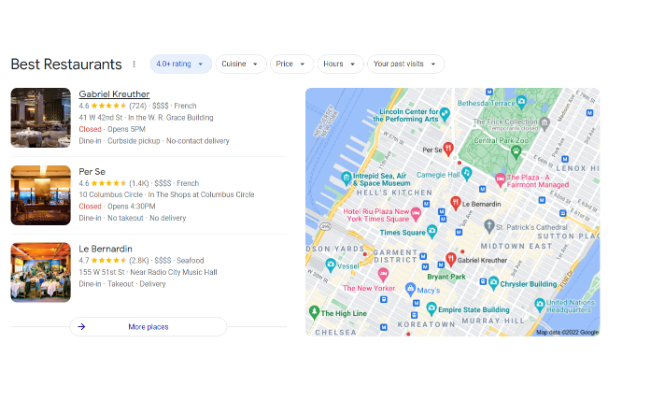The image appears to be a screenshot of a Google search result page dedicated to the best restaurants. The search includes a variety of categories such as cuisine types, price ranges, operating hours, and past visits. The current view is filtered by ratings.

On the right side, there is a map highlighting various neighborhoods in New York City, including Koreatown, Chelsea, Midtown East, and Hell's Kitchen. Numerous location pins are scattered across the map, indicating a high density of restaurants.

At the top of the list of restaurants is Gabriel Kreuther, boasting a 4.5-star rating based on 734 reviews. This upscale French restaurant is marked with four dollar signs, denoting higher prices. Below it is Per Se, another French establishment with the same 4.5-star rating but nearly 1,400 reviews, also listed with four dollar signs. Le Bernardin, yet another highly acclaimed option, stands out with a 4.7-star rating from 2,800 reviews. This seafood restaurant also carries a four-dollar-sign price tag.

All the listed restaurants are highly rated, indicating a quality dining experience, but potential visitors should be prepared for a significant expense.